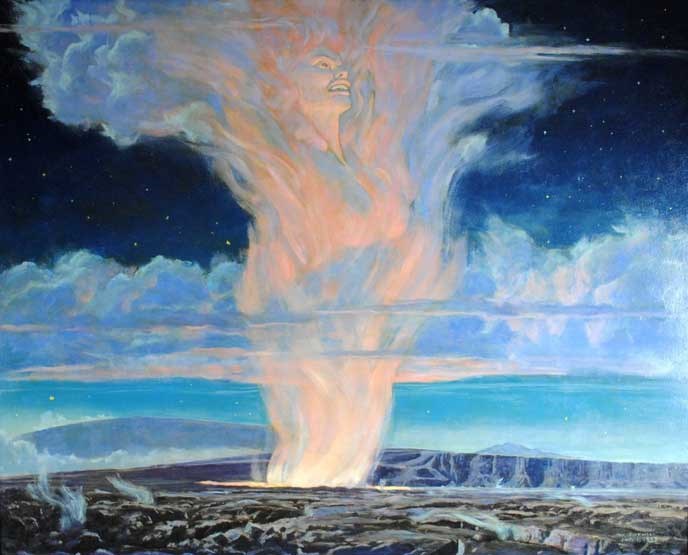In this vibrant, hand-drawn painting, a dramatic plume of smoke ascends from a mountainous landscape, dominating the entire vertical space. The dense smoke is rendered in a mesmerizing blend of red, pink, and orange tones, with hints of yellow, forming the abstract shape of a woman's head near the top, her face a mix of grimacing and smiling expressions. The artwork transitions from an earthy base of browns, grays, and whites, representing the ground and rocks, through layers of atmospheric blue, turquoise, and white clouds. At the very top, the image shifts to an ethereal, star-studded space, epitomizing a dark, almost galactical ambiance. The soft, muted colors and brush strokes contribute to the surreal, mystical nature of this celestial scene.